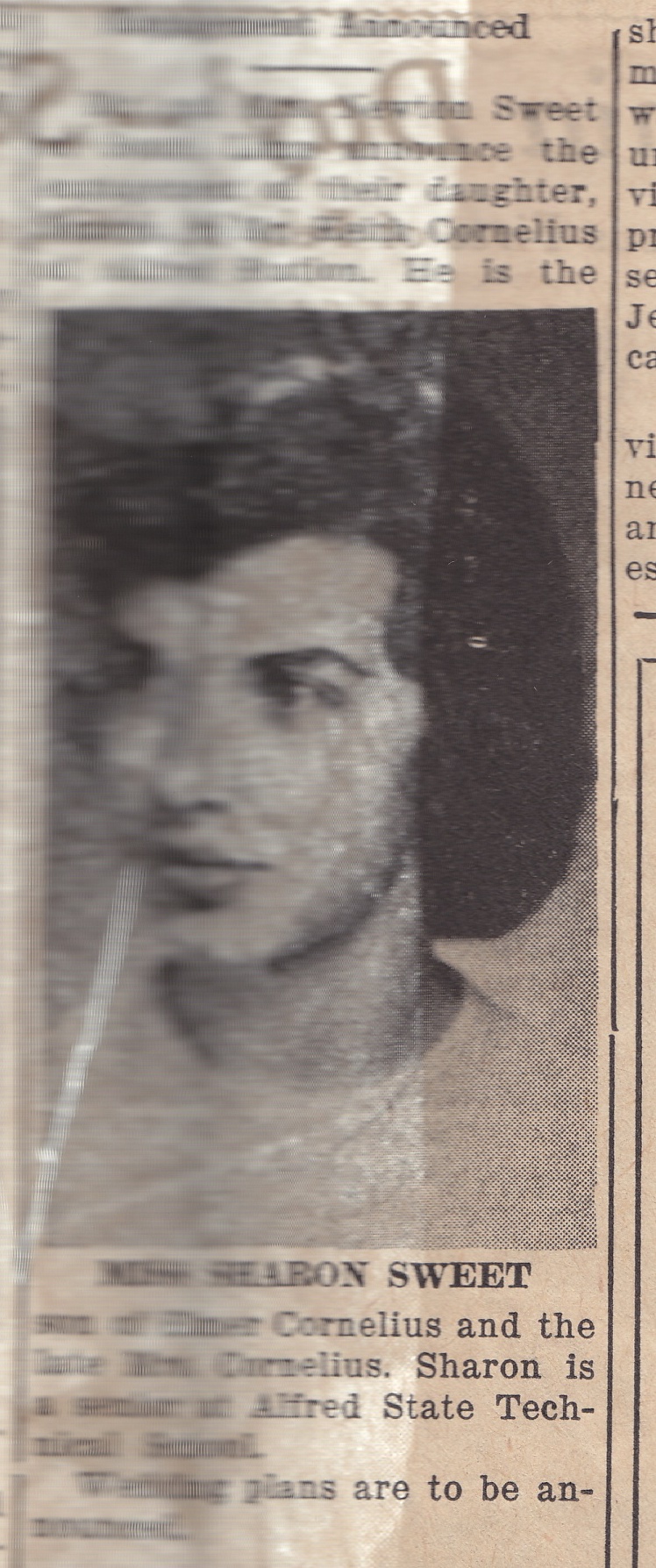This is a photograph of a severely out-of-focus black and white newspaper clipping. The image features a headshot of a young woman with long dark hair, smiling and looking slightly to our left. She is dressed in a light-colored top or dress with a high neckline. The faded text surrounding the image exhibits signs of browning or yellowing, suggesting significant age. There is noticeable glare or shadowing on the right side of the clipping. Although most of the text above and below the photograph is illegible, the name "Miss Sharon Sweet" can be discerned under the image. Additionally, the words "Cornelius," "Sharon," and a few other indistinct terms are partially visible, leading to speculation that this could be related to a wedding announcement rather than an obituary.